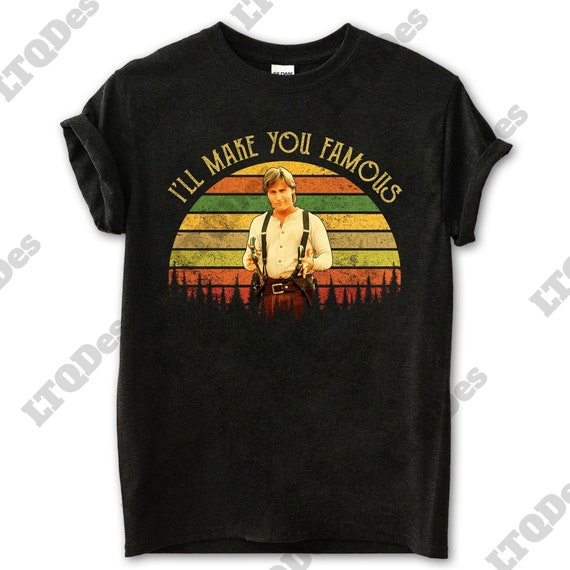This black, short-sleeved t-shirt features a striking design centered around Emilio Estevez portraying Billy the Kid, as depicted in the movie "Young Guns." Estevez, dressed in a white shirt and leathery-looking pants with chaps, also sports suspenders holding up his pants. In each hand, he holds a gun, with holsters attached to his waist. Above Estevez, in bold, capitalized gold letters, the phrase "I'll make you famous" arcs in a semicircular pattern. This semicircle comprises horizontal stripes in colors reminiscent of the Jamaican flag—yellow, orange, green, red, and beige. A black tree line extends from Estevez’s waist, integrating seamlessly into the t-shirt's design. Additionally, the background of the shirt is adorned with a repeating diagonal pattern of the letters L, T, Q, D, E, and S intermittently showing in gray. A white tag is visible at the back of the collar.